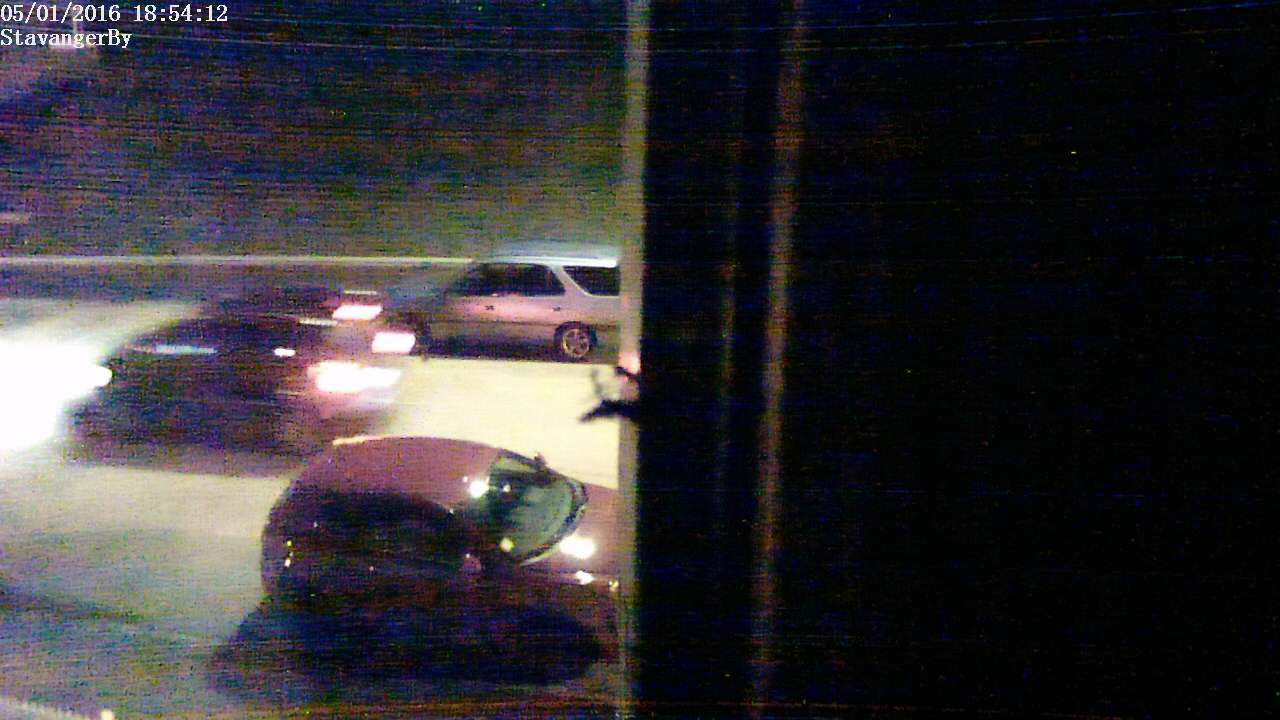This image is a still captured from a security camera, looking out of a partially shuttered window. The shutter on the right-hand side is not completely closed, slightly obscuring the view. Outside, a high red brick wall stands on the opposite side of what appears to be a road or possibly a parking lot. Three cars are visible: a red car and a silver car, which seem to be parked, and a black car with illuminated red brake lights, suggesting it is in motion. The scene is somewhat fuzzy and low-quality, making further details unclear but hinting at a nighttime setting due to visible car lights. A timestamp at the top of the image reads either January 5th or May 1st, 2016, recorded at 16:54 or 18:54, and includes the text "Stavanger Bay."